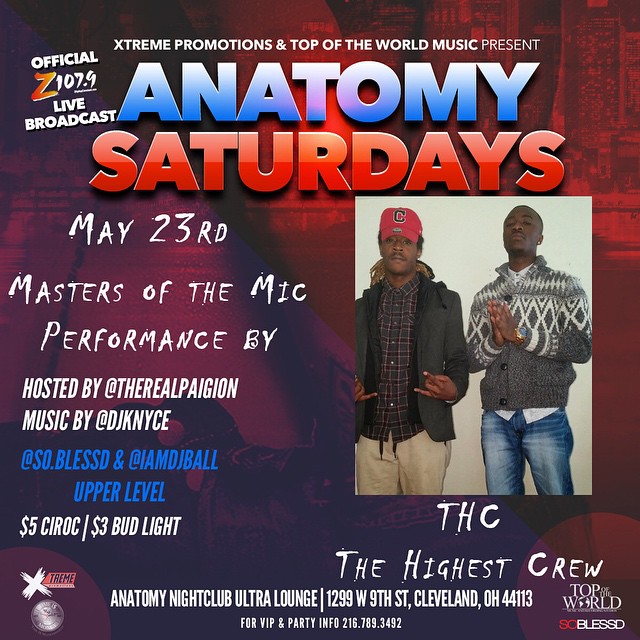This digital promotional flyer advertises "Anatomy Saturdays," an event presented by Extreme Promotions and Top of the World Music. The title is prominently displayed with "Anatomy" in bold blue text fading from light to dark, and "Saturdays" in bold red text with a gradient from pale red to dark red. The background features a dark red wall-like texture. 

At the top, in small white letters, it reads "Extreme Promotions & Top of the World Music Present." Below this, "Official Z107.9 Live Broadcast" is noted on the far left. 

The event is scheduled for May 23rd, as indicated in a handwritten-style font. Billed as "Masters of the Mic," the performance lineup includes hosts and DJs such as The Real Paigion, DJ Knyce, So Blesso, and I Am DJ Ball. These names are written in varying fonts that suggest a handwritten look.

In the middle right section of the flyer, there's a photograph of two musicians. The man on the left, wearing an orange baseball cap with a "C" and a dark plaid shirt with a jacket, has his hands forming a gang symbol. The man on the right, dressed in a gray sweater with a white diamond pattern and blue jeans, holds his hands clasped in a prayer-like pose. This image is labeled "THC, The Highest Crew."

Pricing details are also included: "$5 Ciroc," "$3 Bud Light." At the bottom of the flyer, the location is given as "Anatomy Nightclub Ultra Lounge, 1299 West 9th Street, Cleveland, Ohio 44113." For VIP and party info, the contact number provided is 215-783-3492. The lower section of the flyer also displays logos for Top World and So Blesso.